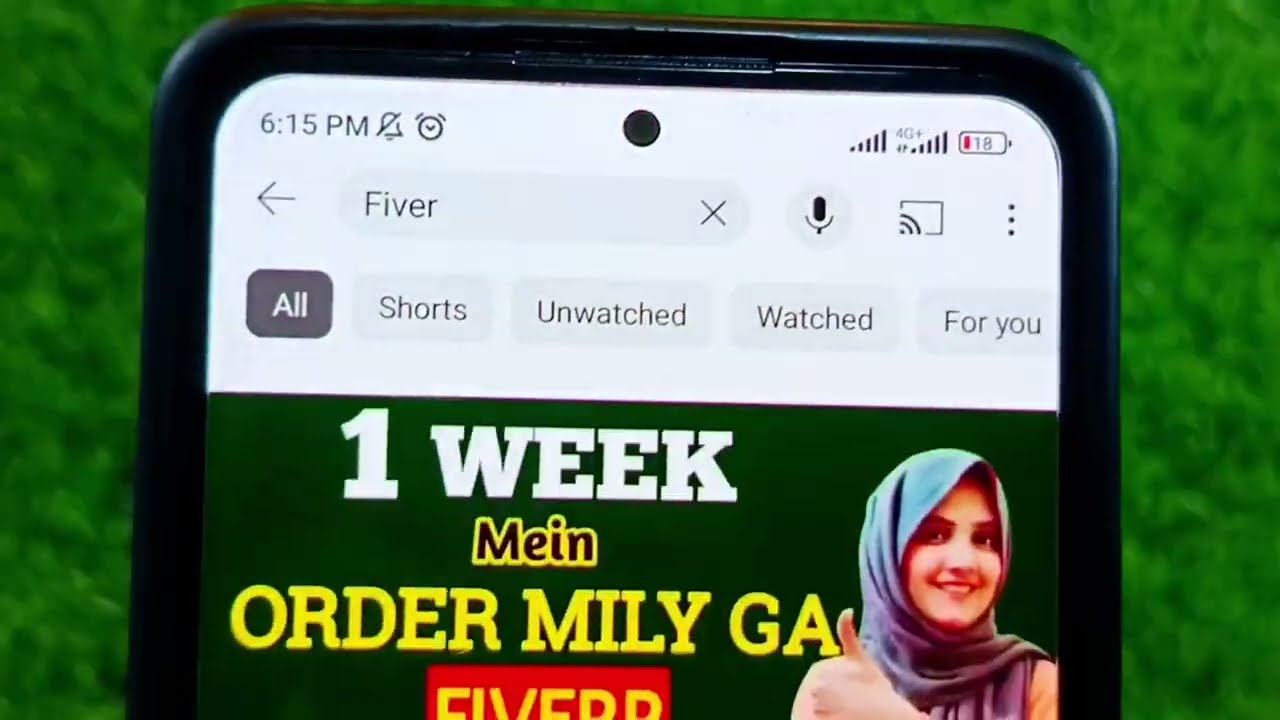This close-up color photograph showcases a black-edged smartphone with a blurred green grassy background. Displayed on the phone screen, the status bar indicates various icons: the clock showing 6:15 PM, a crossed-out bell symbol (indicating muted alerts), an alarm clock icon, a 4G+ signal indicator, and a battery level at 18%. The top of the screen features a search bar with "Fiverr" typed in. Below the search bar, tabs labeled "All Shorts," "Unwatched," "Watched," and "For You" suggest a YouTube-like interface. The central section of the screen shows a video thumbnail depicting a smiling woman wearing a hijab, accompanied by text reading "One Week Main Order Miley GA Fiverr," along with a thumbs-up icon.